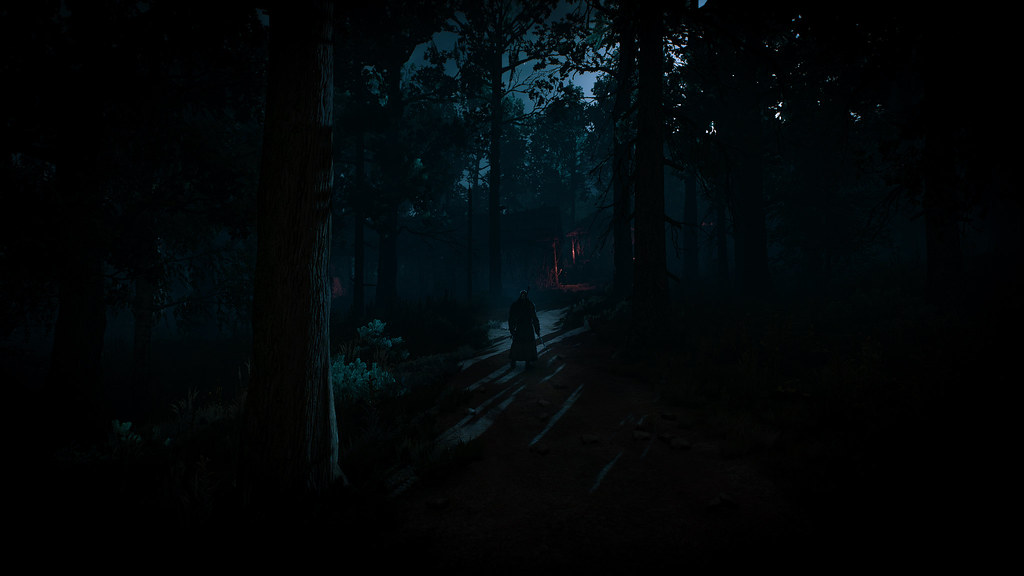In this image—which is either a painting or a screenshot from a video game—we see a haunting nighttime scene set in a very dark, densely wooded forest. The dominant colors are dark blues and blacks, creating a deeply shadowed atmosphere. Toward the center of the image, a silhouetted human figure walks along a path, seemingly heading towards a faintly glowing red-orange light that might represent a small cabin or a fire. The figure appears to be holding a long, pointy object, possibly a sword, and is dressed in a long coat or jacket. Large trees and thick bushes surround the path, their details subtly revealed by dappled moonlight filtering through the canopy. The moon itself, a light periwinkle blue, peeks through the leaves, casting an eerie glow over the scene. The edges of the image are enveloped in darkness, enhancing the ominous, sinister mood of the setting.